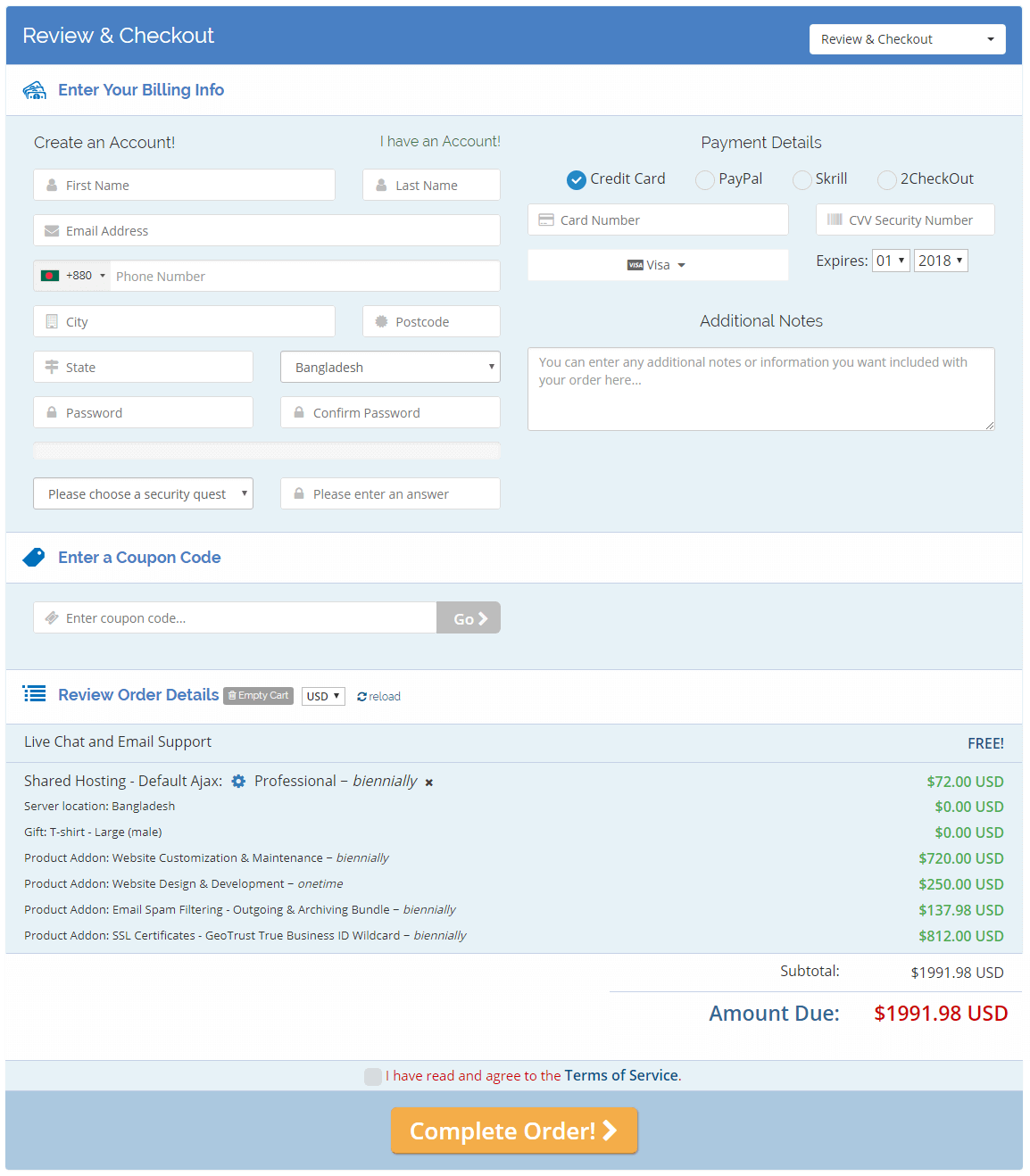A detailed and polished caption for the image could be:

"The page displayed is titled 'Review and Checkout' and features a prominent blue border. It prompts users to enter their billing information, complete with a search bar and a drop-down menu for detailed entries. The form includes fields for creating an account, asking for First Name, Last Name, Email Address, Phone Number, City, State, and Country, all with drop-down options. There are boxes to enter and confirm your password, followed by a prompt to select a security question. The page also contains sections for reviewing order details, offering live chat and email support options. Further down, the page is slightly blurry but lists 'Payment Details' where users can choose between Credit Card and PayPal payment methods. It includes fields for Card Number and CVV security code, along with a section for additional notes accompanied by a text box for user input."